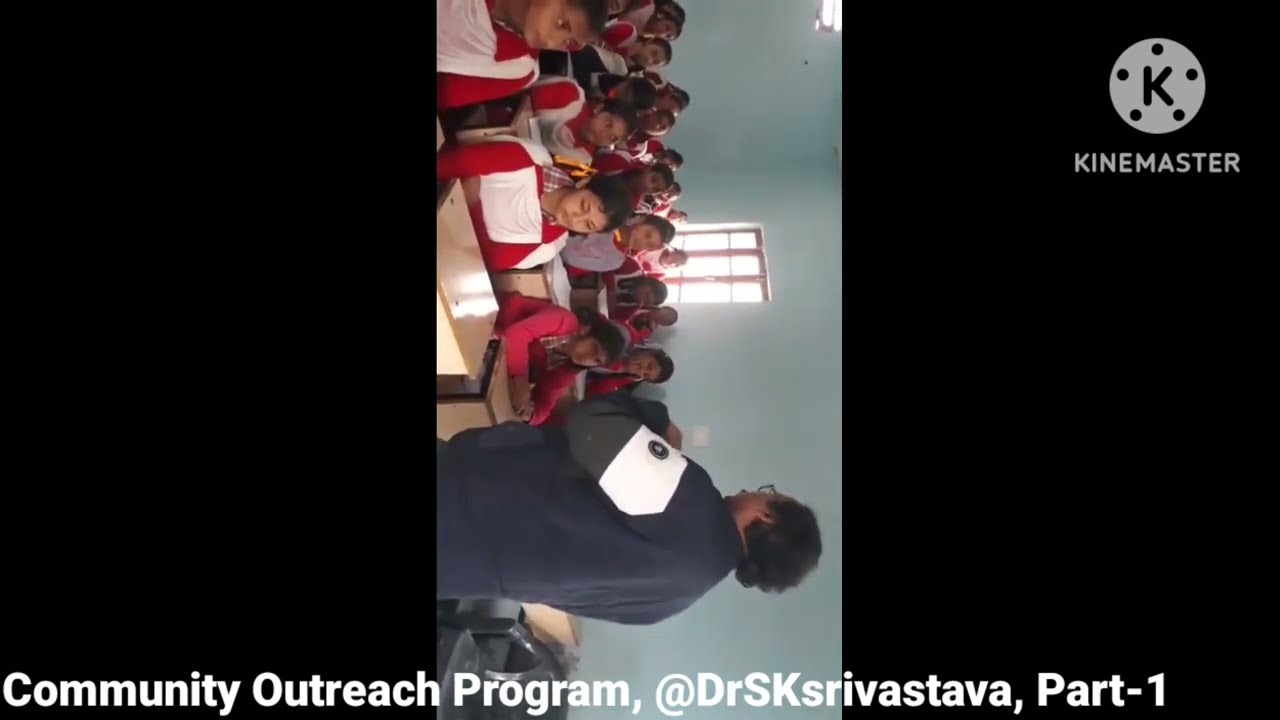The image is a horizontally oriented rectangle divided into three equal sections. Both the left and right sections have black backgrounds. The right section features a logo in the upper right corner, consisting of a circle with the letter "K" at the top, and the word "KINEEMASTER" beneath it. In contrast, the middle section displays a rotated photograph of a classroom, which appears to be set in India. Centrally featured in this section is a man with medium-length black hair and glasses, wearing a blue shirt with a white armband. He stands at the front of the room, presumably teaching, while multiple young girls, with light brown skin and black hair, clad in red and white uniforms, sit attentively at their small wooden desks. The classroom has a white wall with a single window at the back, allowing light to stream in. Across the bottom of the entire image is a text in white letters, reading: "COMMUNITY OUTREACH PROGRAM, @drsksrivastava, part-1."